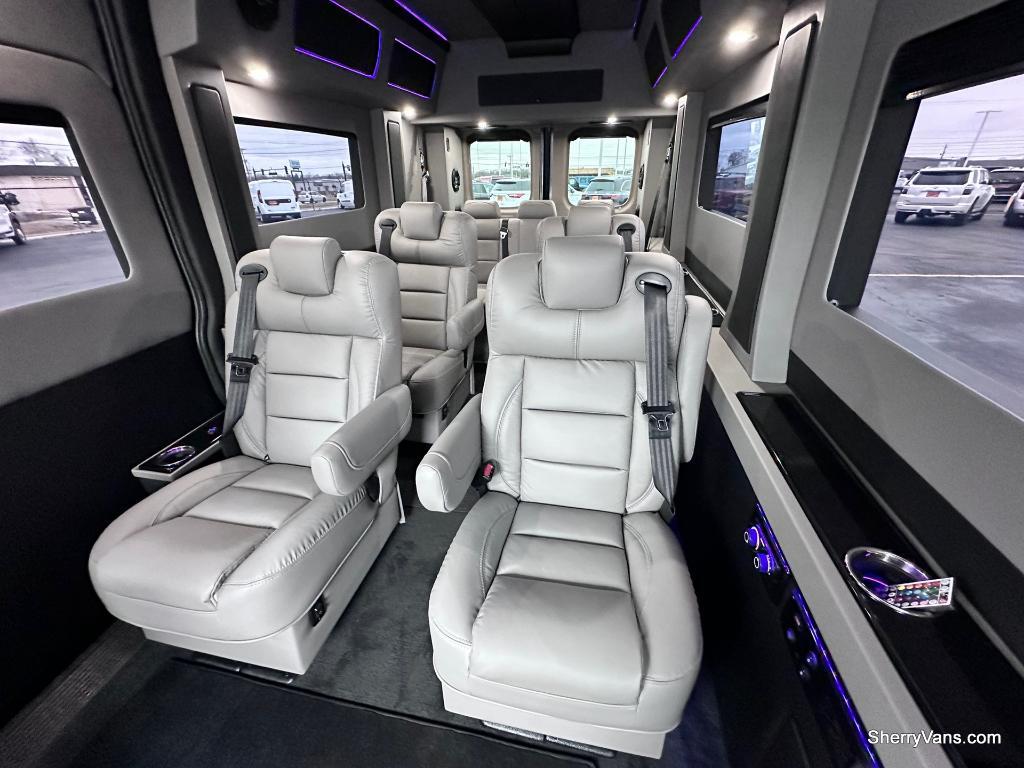The image shows the interior of a spacious, luxury passenger vehicle, resembling a high-end van or limousine, with several notable features. The seats are upholstered in pristine white leather, arranged in two rows of individual bucket seats with armrests and cup holders, followed by a rear bench seat that can accommodate three passengers. This setup allows for a comfortable seating capacity of up to seven people. Each seat is equipped with a gray seatbelt for safety. The vehicle's interior is illuminated with ambient purple lights that add a touch of elegance, particularly around the black cup holder areas. The floor is covered with a gray rug that complements the white interior. On the right side, there is a compartment holding a remote. Windows line the sides and back of the vehicle, providing a clear view of the outdoor parking lot, where other vehicles such as a white car and a white van can be seen. The bright daytime setting enhances the clarity of the image, and in the bottom right corner, the website "SherryVans.com" is visible, indicating the vehicle's likely manufacturer or dealer.